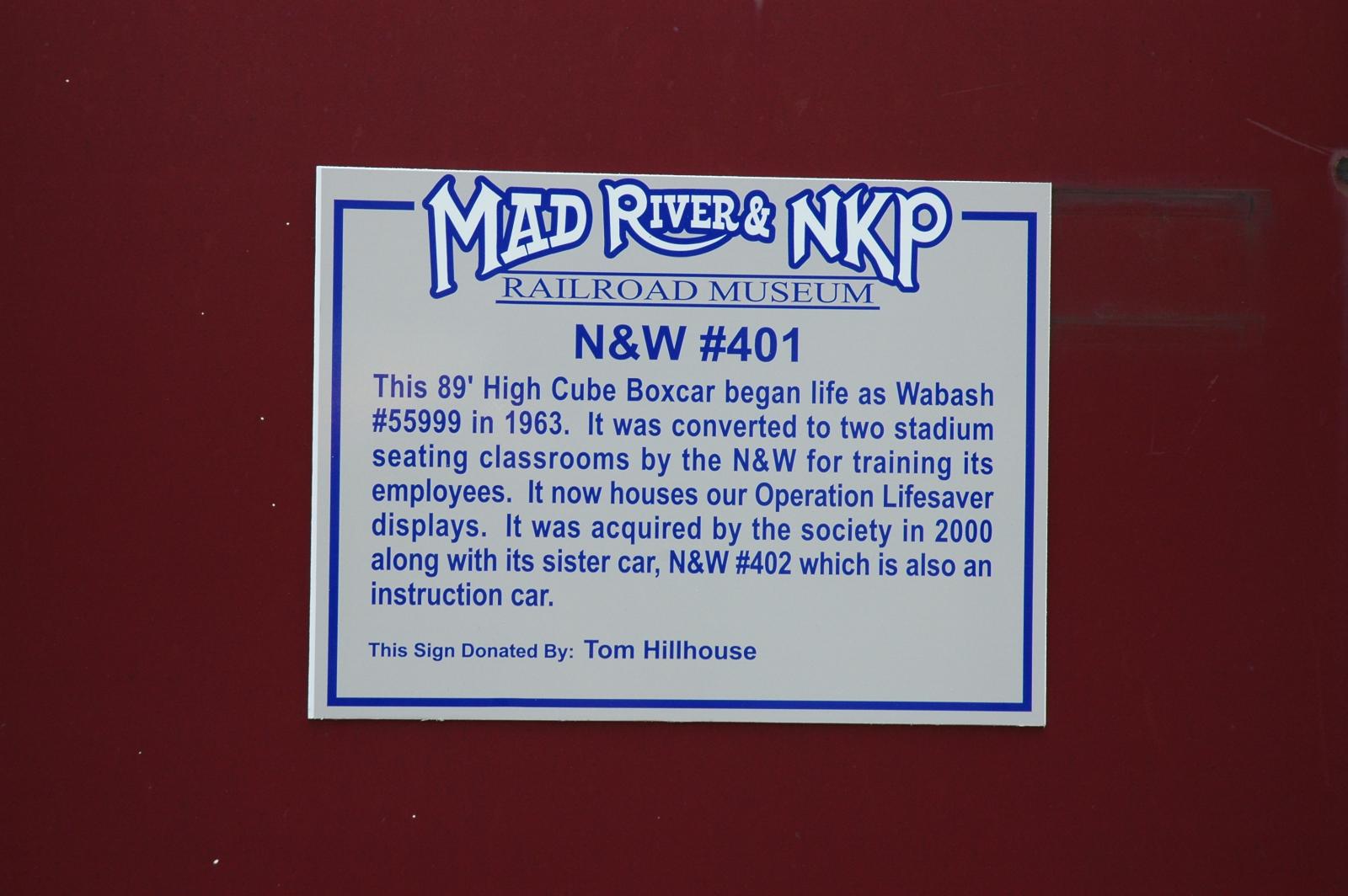The photograph depicts an extreme close-up of a railroad car colored in a dark, rusty burgundy hue, typical of railcars. The focal point is a gray rectangular sign, bordered by a dark blue outline, prominently displayed in the center of the image. Across the top of the sign, bold white lettering reads "Mad River and NKP", followed by blue text stating "Railroad Museum." Below, it identifies the railcar as "N&W number 401." The detailed description on the sign reveals that this 89-foot high cube boxcar began its life as Wabash number 55999 in 1963. It was later converted by the Norfolk & Western (N&W) into two stadium seating classrooms for training employees. The car now houses Operation Lifesaver displays and was acquired by the Society in 2000, along with its sister car, N&W number 402, which is also used for instruction. The sign concludes with the note, "This sign donated by Tom Hillhouse."